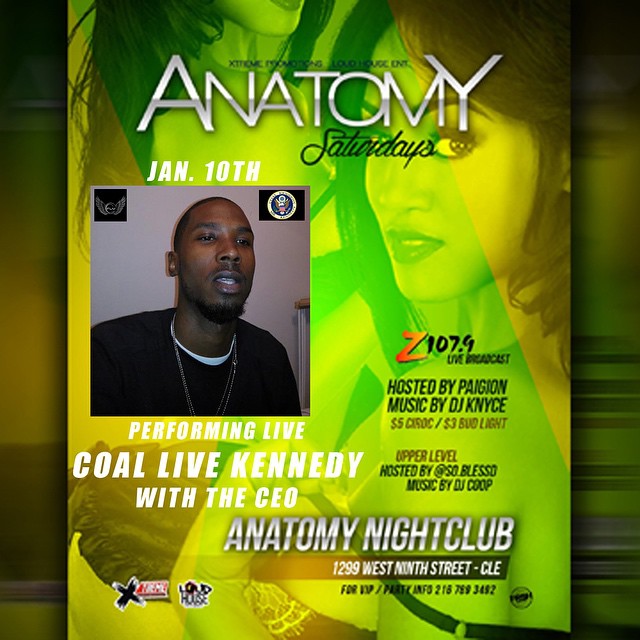The image is a lime green and green advertisement for a concert or meet-up event at Anatomy Nightclub. Dominating the top of the poster, large white letters spell "Anatomy", with "Saturdays" in black script font just beneath. The event is scheduled for January 10th and prominently features a photograph of a man in a black t-shirt wearing two necklaces, with his mouth open as if he is talking. This man is performing live as "Co-Live Kennedy with the CEO". Below his image, in white letters, there's the detailed information about the event being a Z107.9 live broadcast, hosted by Paigon with music by DJ Nice. The venue, Anatomy Nightclub, is located at 1299 West 9th Street, CLE. Faded, translucent images of women provide a subtle background element. The lower part of the poster lists the price of alcohol and other contact details.